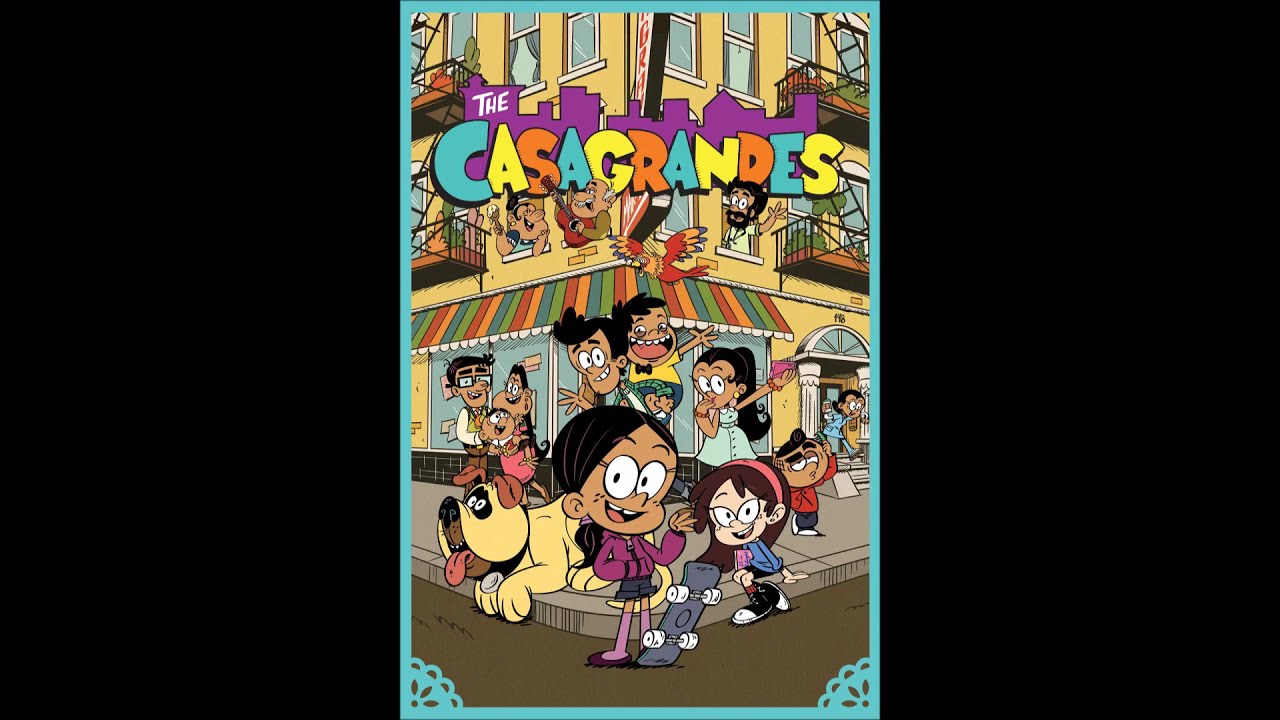Centered within a black border, the vertical cartoonish poster vividly portrays a bustling, colorful street scene with a whimsical and lively atmosphere. At the top, in white letters, are the words "The Casa Grandes," with "Casa Grandes" spelled out in alternating bright colors: blue, yellow, and orange, set against a light blue cityscape skyline. The central focus is a diverse group of cartoon characters in front of a striped-awning corner store. 

In the foreground stands a smiling young girl with large eyes and dark hair in a ponytail, wearing a purple jacket and holding a skateboard. Beside her on the left is her friendly yellowish dog, tongue hanging out. Surrounding her are other characters, including a girl with a headband sitting on the curb, a little boy in red, and another girl dressed in white. Additionally, a man with a beard and glasses carries a smiling child on his shoulders behind them. 

Above and within the building, various characters interact with their surroundings: people lean out of windows, including a man playing a guitar and another waving enthusiastically. The vividly detailed backdrop includes features like fire escapes, balconies, and a vibrant, colorful overhang. The entire image radiates a sense of community and animated joy, emphasizing the dynamic and friendly environment of "The Casa Grandes."